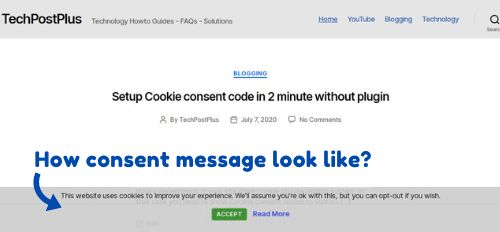This image is a slightly blurry screen capture of a website, identified by the gray bar at the top which reads "Tech Post Plus" in black text. This bar also contains the site’s various sections: "Technology," "How-to Guides," "FAQs," and "Solutions." The right side of the gray bar features clickable blue text links labeled "Home," "YouTube," "Blogging," and "Technology," alongside a gray magnifying glass icon.

Scrolling down, the heading "Blogging" appears in blue, followed by a black text subheading promising a tutorial: "Set up cookie consent code in two minutes without a plugin." Below this, in gray text, the article is credited to "Tech Post" and a name that looks like "plan," accompanied by a small head and shoulders icon. Next to this, a calendar icon shows the date "July 7th, 2020," and a text message icon indicates "no comments." 

In blue, a subheading "How consent messages look like" introduces a section where a gray box displays a standard cookie consent notification: "This website uses cookies to improve your experience. We'll assume you're okay with this, but you can opt-out if you wish." This message is followed by a green button labeled "Accept" in white font and a blue "Read More" link beside it, all somewhat blurred and slightly warping.

Overall, the image is slightly smudged and blurred, which affects the clarity of the text and icons. This blurred effect gives the screen capture a smudgy, unfocused appearance, with no other significant details noteworthy for further analysis.